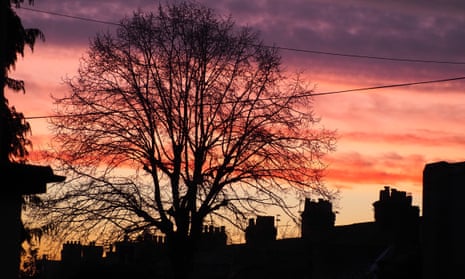A horizontal, rectangular photograph captures an evocative scene either shortly after sunset or just before sunrise. Dominating the foreground is a tree, mostly appearing in shadow, its thin, leafless branches spread throughout the image, forming a hemispheric shape. The dark silhouette of the tree, with its trunk splitting into four or five main branches, contrasts strikingly against the vivid, streaked sky. The sky transitions from gray and white at the horizon, progressing through hues of orange and light pink midway, to deeper shades of purple and pink higher up, highlighting the setting or rising sun. Multiple rows of nearly identical buildings with rectangular forms and multiple antennas or smokestacks emerge faintly in the background, suggesting a factory-like structure. Black cables, likely electrical wires or telephone lines, extend horizontally from the left to the right side, cutting across the image. An evergreen tree silhouette is visible along the left side, adding to the depth and complexity of the scene.